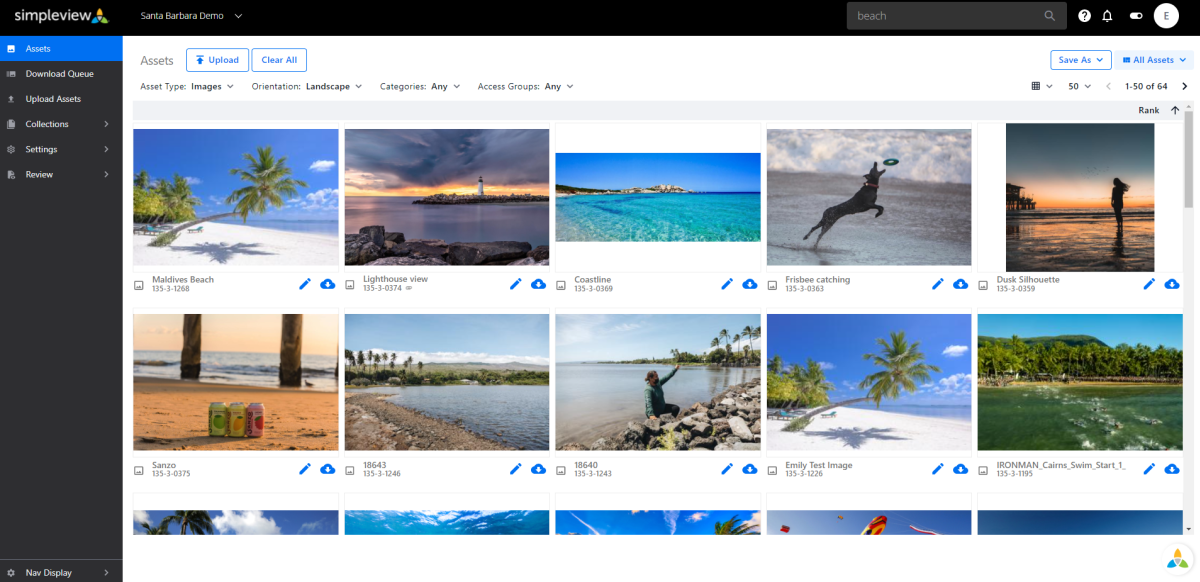The screenshot displays the interface of the Simple View app. The top-left corner features the Simple View logo. Along the left side of the page runs a very narrow vertical black panel, while a similarly narrow horizontal black header spans across the top. The main body of the page has a white background.

Within the main body area, photo thumbnails are organized in horizontal rows. Each thumbnail includes specific information: the bottom left corner shows the location and date the photo was taken, and the bottom right corner features a blue pencil icon for editing and a blue cloud icon for other actions.

Above these thumbnails, on the left side, there are various filter options: "Asset Type" with a dropdown box set to "Images," "Orientation" set to "Landscape," "Categories" set to "Any," and "Access Groups" also set to "Any." 

On the far right, another dropdown box is set to display 50 items per page. Adjacent to this dropdown, there are page navigation controls, indicating "Page 1-50 of 54," with arrows on either side for moving forward or backward through the pages.